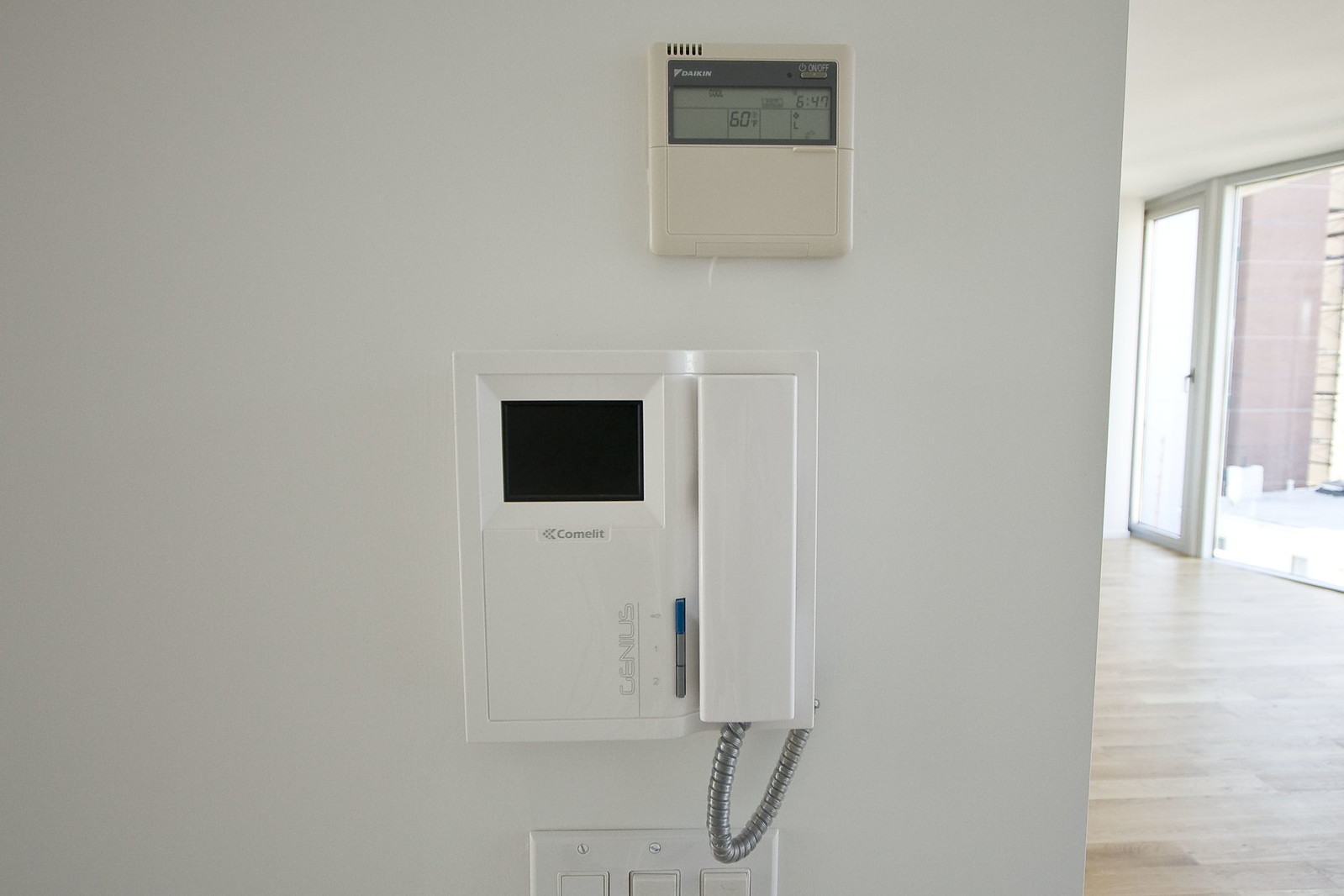The image captures the interior of a house, showcasing a section of a white wall adorned with several electronic devices. At the top of the wall is a cream white thermometer with a grayish screen and gray outline, displaying the number "60," which could represent either the temperature or humidity level. Directly below the thermometer is a white doorbell featuring a black screen. Beneath the doorbell, a set of switches is visible. In the corner, a glass sliding door can be seen, allowing an ample amount of natural light to flood the space. The floor beneath these features is polished and adds a touch of elegance to the room.